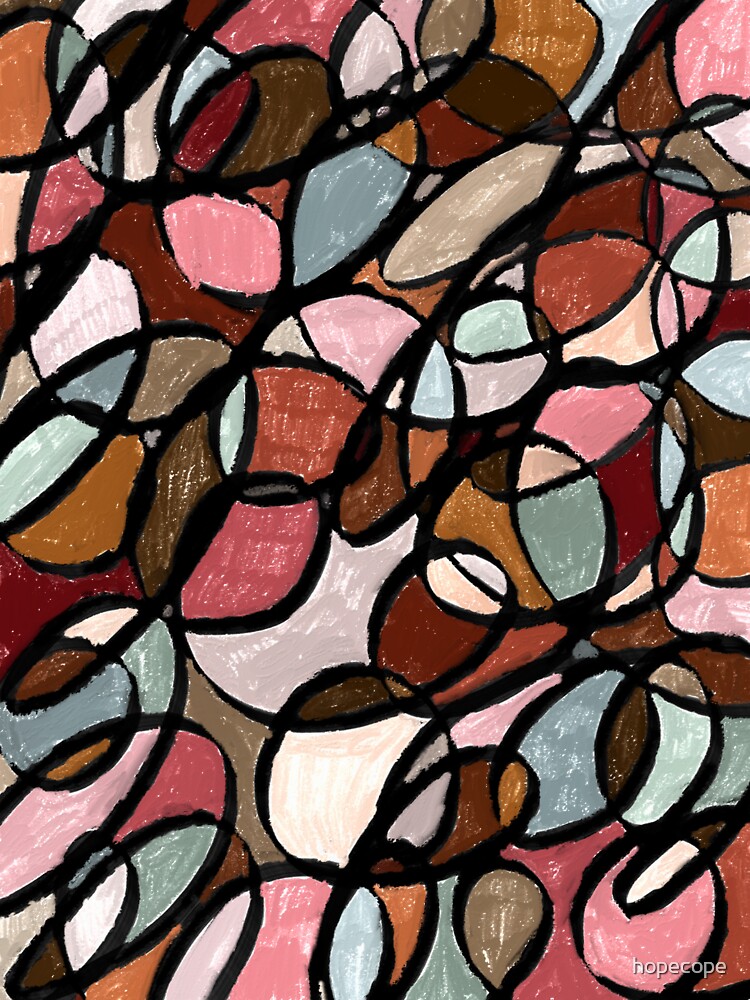This vertically oriented, abstract painting embodies a stained-glass-like effect with its interlocking geometric shapes, primarily ovals, circles, and semicircles. Signed "hope cope" in lowercase white letters at the bottom right corner, the piece features thick, black outlines that bisect and intertwine the myriad shapes, creating intricate panels. The rich, pastel color palette includes pink, orange, brown, blue, gray, and mauve, arranged such that no two adjacent shapes share the same color. Resembling paintbrush strokes, light specks add texture, giving the impression of watercolor or pastel oils. The painting is a harmonious blend of earthy and vibrant hues, presenting a captivating and detailed composition devoid of any additional border.